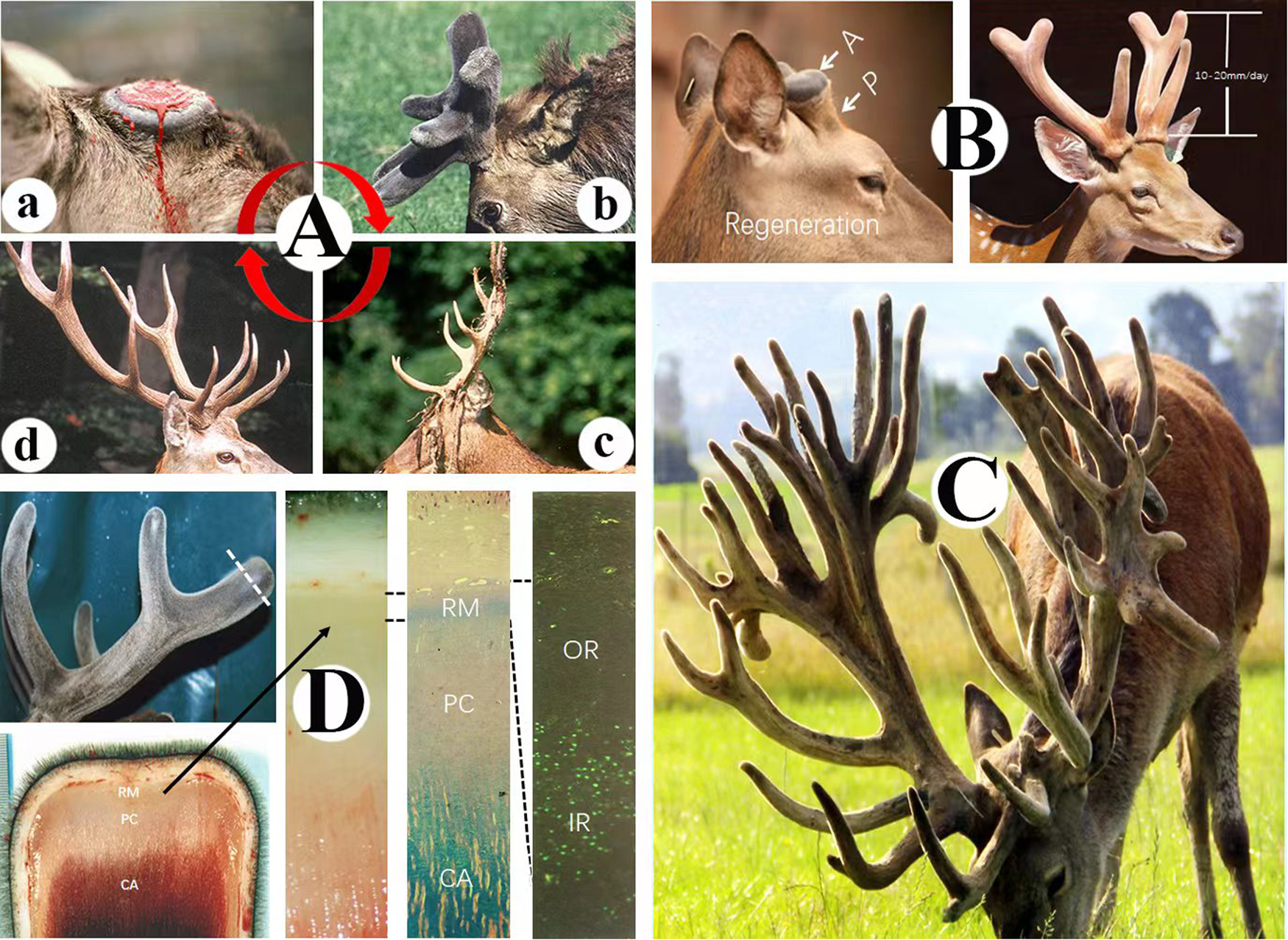The image is a detailed, landscape-oriented diagram consisting of approximately eight to ten color photographs and illustrations, focusing on the different stages of deer antler development. Each section is labeled with a letter inside white circles with black text, aiding in the educational clarity of the visual layout. The topmost section features four smaller images, all labeled "A," depicting early-stage antlers. Adjacent to this, there are two side-by-side images labeled "B," showing a deer head both with and without antlers. Below these, a larger image labeled "C" showcases a full-bodied deer with an exaggerated set of mature, possibly digitally modified antlers, which might represent a 25 or 30-point buck. The leftmost section, labeled "D," includes detailed illustrations of cross-sections and mid-development antlers, accompanied by arrows and other graphic elements to highlight specific parts and stages. This compilation, blending photographic realism with illustrative elements, serves as an educational tool to describe the scientific process of antler growth and development in deer.